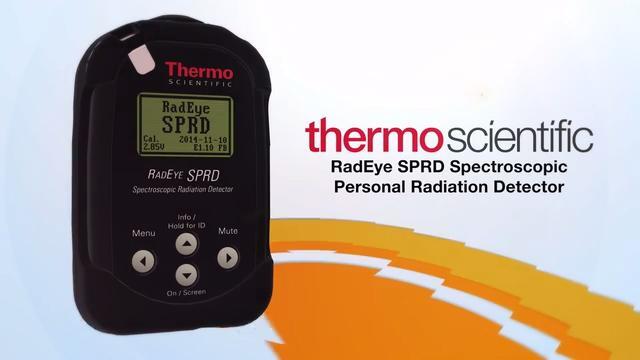The image appears to be an advertisement set against a predominantly off-white and light gray background. On the right side, prominently in red text, it reads "Thermo." Below this, in black text, it says "RedEye Spectroscopic Personal Radiation Detector." There are orange and white lines forming a patch-like design that starts at the bottom right and stretches diagonally across, intersecting with the product itself. The featured product is small and black with white arrow buttons, marked with black arrow points, at the bottom. Below these buttons, "ON/SCREEN" is inscribed in white. The device also has a green screen displaying "RedEye SPRD" in black text.